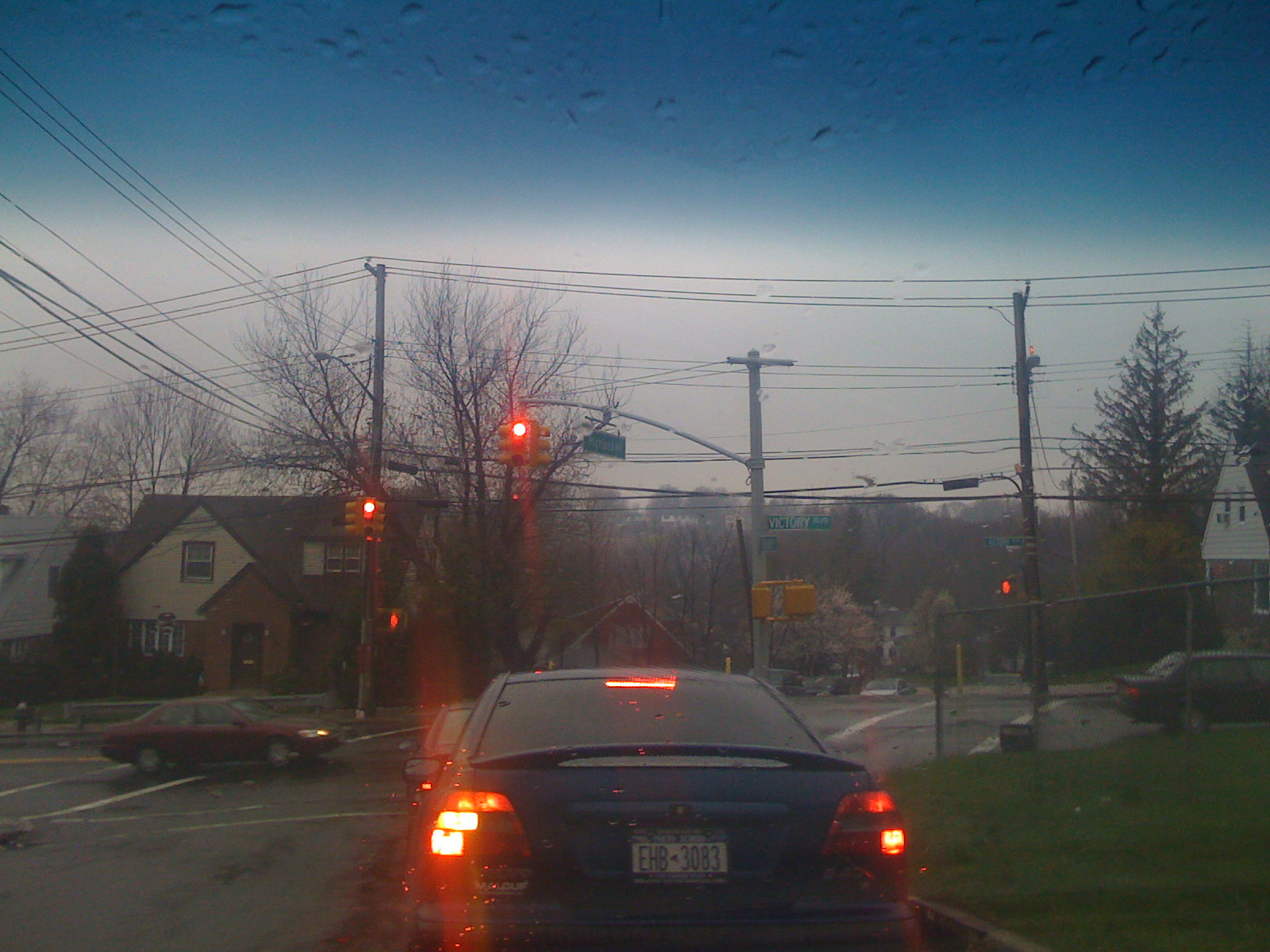This image captures a rainy intersection from the perspective of someone sitting inside their car, looking out through the front windshield at a red light. Directly ahead, a small blue car with a blurry white and blue license plate and illuminated brake lights waits at the intersection. The windshield shows raindrops, with a clear streak in the middle indicating the wipers have recently cleared away the rain. Through the left side of the frame, a maroon sedan passes through the intersection in the cross traffic, signifying it has the green light. In the background, a house sits on the corner, framed by numerous electrical wires and poles, while a hill rises in the distance beneath a cloudy, blue-gray sky. To the right, another car can be seen heading out of the intersection, moving to the right edge of the image. Pedestrian crossing lines are visible on all three sides of the intersection, and sparse, leafless trees hint at a winter setting. Grass patches are noticeable to the right, adding a splash of greenery to the otherwise subdued scene.